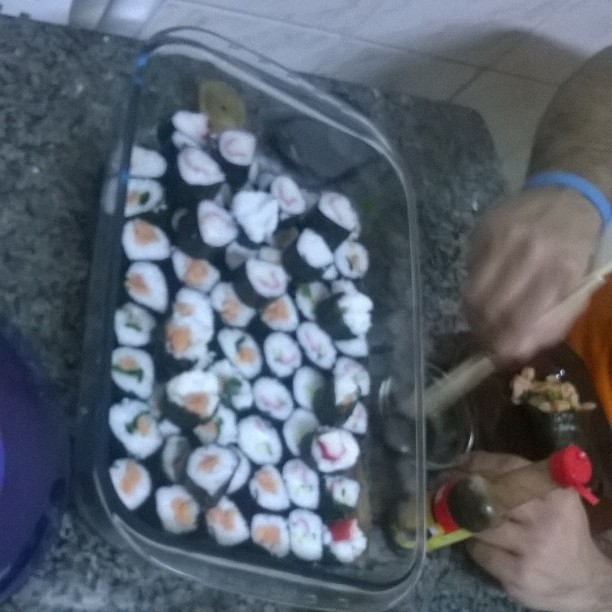This image depicts a somewhat blurry and dimly lit scene with a man, identified by a blue bracelet on his right wrist, holding chopsticks and stirring or dipping them into a small glass bowl of soy sauce. Positioned in front of him is a large rectangular Pyrex baking dish, approximately 9x13 inches, filled with neatly rolled maki sushi. The sushi rolls, wrapped in seaweed, contain a variety of fillings including tuna, crab, and possibly other seafood and vegetables, adding vibrant splashes of yellow, green, and pink to the scene. The dish rests on a granite or marble countertop with a stone-like finish. Beside the glass dish is a clear soy sauce bottle with a red cap and a yellow label. The background features a wall covered in white tiles, enhancing the overall kitchen setting. This detailed visual captures a moment of culinary preparation or enjoyment, focusing on the sushi, soy sauce, and the ambiance of the tiled kitchen.